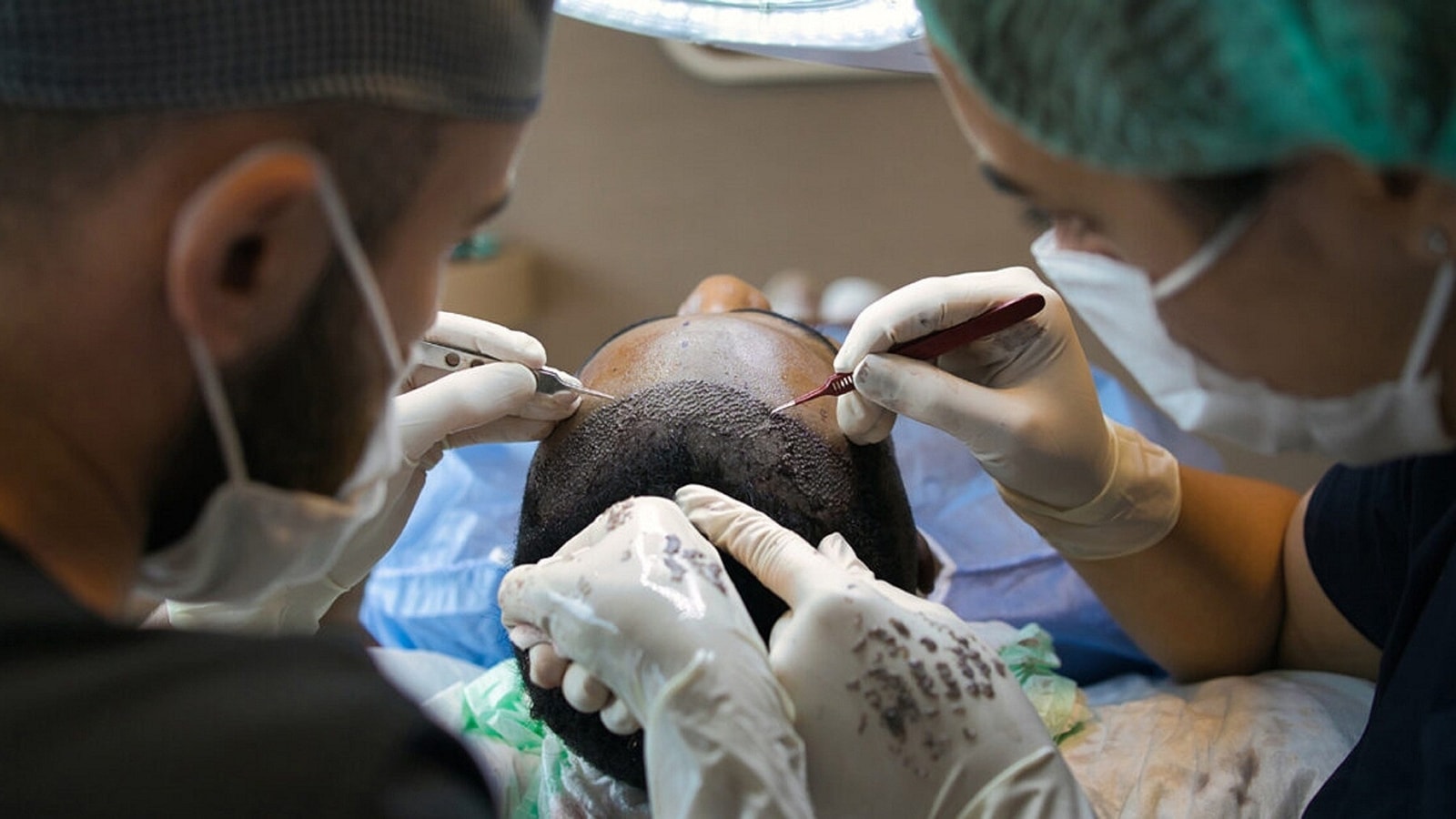In this detailed surgical scene, captured from the perspective over the doctors' shoulders, a hair transplant procedure is underway. The patient, a black male, lies on a gurney, clad in a blue gown. The viewpoint offers a clear look between two medical professionals – the doctor on the left, a bearded man, and the doctor on the right, likely a woman, both outfitted in green scrubs, white face masks, hair covers, and gloves. They are meticulously working on the top of the patient's scalp, where the man's hairline appears bloody, indicative of the transplantation process. Tiny needles and sharp medical instruments, held delicately in their hands, are used to implant hair, with visible hairs scattered across their gloves. Above, a surgical spotlight casts a bright light over the focused activity. The collective effort aims to reconstruct and improve the patient’s hairline, suggesting a precision-focused, collaborative medical endeavor.